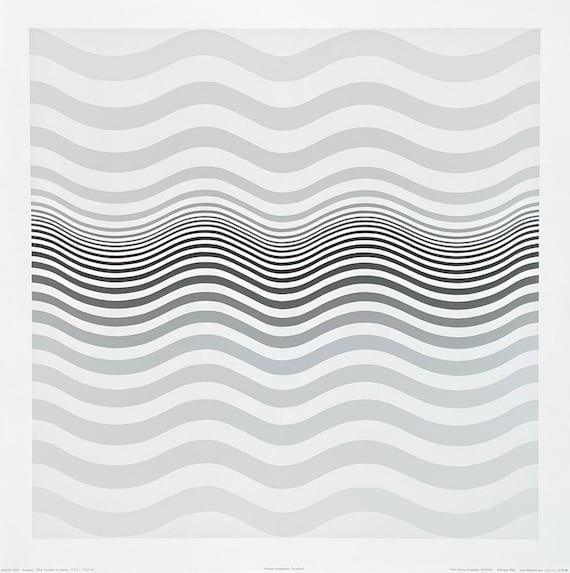This captivating art print, largely monochromatic with a focus on varying shades of gray and minimal black, features an abstract and mesmerizing wave pattern. Set within a narrow grayish-white border, the image consists of repeated, symmetrical horizontal waves that span from top to bottom. The top portion of the image showcases thicker, lighter gray waves against a white background. As the pattern descends towards the middle, the waves become thinner and darker, converging closer together, and reaching a near-black color. This gradient shift continues downwards, with the waves broadening once more and lightening back to a pale gray, mirroring the top section's width and shade. This wave pattern, consistent and continuous, evokes a visual illusion of motion. Additional detail includes unreadable tiny text along the bottom edge of the image, suggesting it is a professional print or photograph of a larger work. The image's symmetry and simplicity, combined with its intricate variance in line thickness and color intensity, create an entrancing and professional piece of abstract art.